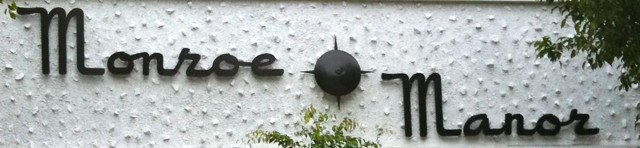A horizontally-oriented photograph features a textured white wall adorned with small protruding bumps. Elegant cursive writing appears on the wall; "Monroe" is inscribed at the top left, and "Manor" at the bottom right. At the center of the wall is a distinctive, round black object decorated with sharp, pointed extensions radiating from its top, bottom, and the middle of its left and right sides. Just below this central object, the tips of a small bush or shrub are visible, revealing lush green leaves. In the right corner of the image, some additional greenery is evident, showing leaves from a nearby tree in the vicinity.